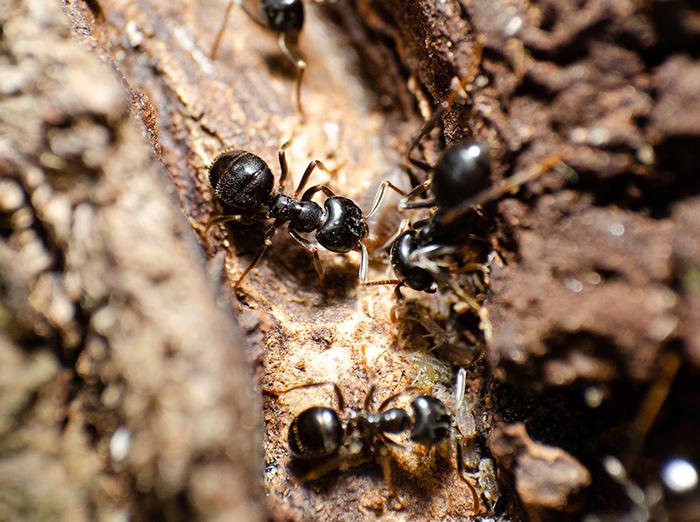The image captures an extreme close-up of four shiny black ants situated against a dark brown background, likely indicating a tree trunk or soil. The ants, each possessing six legs and two antennae, are shown on a surface that ranges in color from beige to brown. The ants exhibit a glossy appearance due to sunlight reflecting off their bodies, suggesting they are in a brightly lit environment, possibly on a sunny day. The focal point of the image is two ants in the center, flanked by clusters of soil-like substances. One ant, prominently positioned in the middle, displays a distinct body structure with a rounded abdomen, a slender midsection, and an identifiable head with antennae. This detailed composition highlights the ants’ activities as they climb over what seems to be bark, emphasizing the intricate and dynamic nature of these small creatures in their natural habitat.